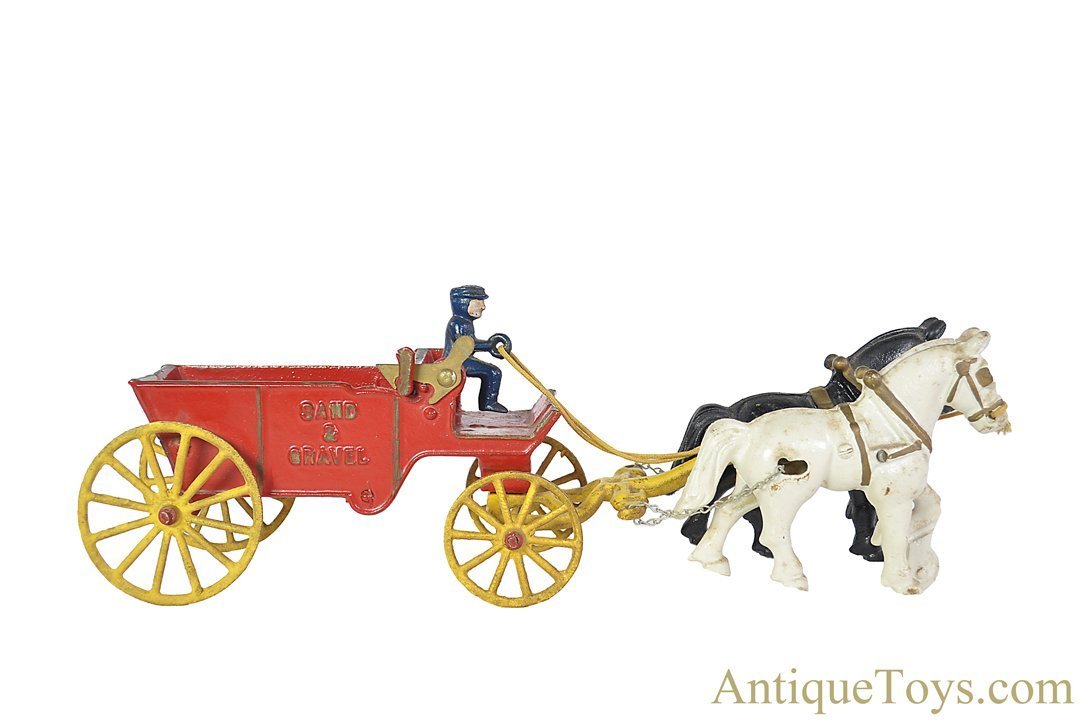This detailed image captures an antique toy depicting a horse-drawn cart or chariot, crafted primarily from metal, possibly with some plastic elements. The setup features two horses at the front—a white horse adorned with golden straps and harnesses, and a black horse similarly outfitted in gold. Both horses are tethered to a vividly red cart marked with the words "Sand and Gravel," which has gold wheels, with larger wheels at the back and smaller ones at the front. The connection between the horses and the cart is highlighted by a gold connector and thin silver chains. Seated at the front is a tiny figure dressed in blue, holding yellow reins, adding to the authenticity of the scene. The overall composition is set against a white background, with “antiquetoys.com” inscribed in the lower right corner. The toy's elaborate details and classic design evoke a nostalgic glimpse into yesteryears.